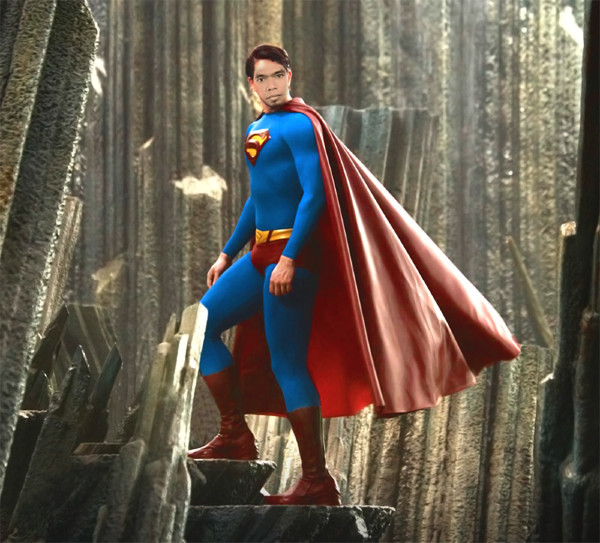This is a detailed, computer-generated image of a man dressed as Superman, though his face has been photoshopped with a different, possibly Asian, face that doesn’t anatomically fit the body and appears slightly too small. The character wears the traditional Superman costume: a blue leotard, a yellow and red belt, red shorts, red boots, and a long flowing red cape, emblazoned with the iconic Superman logo on the chest. He stands on some rocks within an ambiguous background that combines elements of a forest with sunshine and fallen trees, yet also suggests the crystalline structures of the Fortress of Solitude. The lighting in the image is inconsistent, with odd shadows, particularly a pinkish one on the right side of the face. The overall composition is dramatically flawed, giving it a comical and surreal effect.